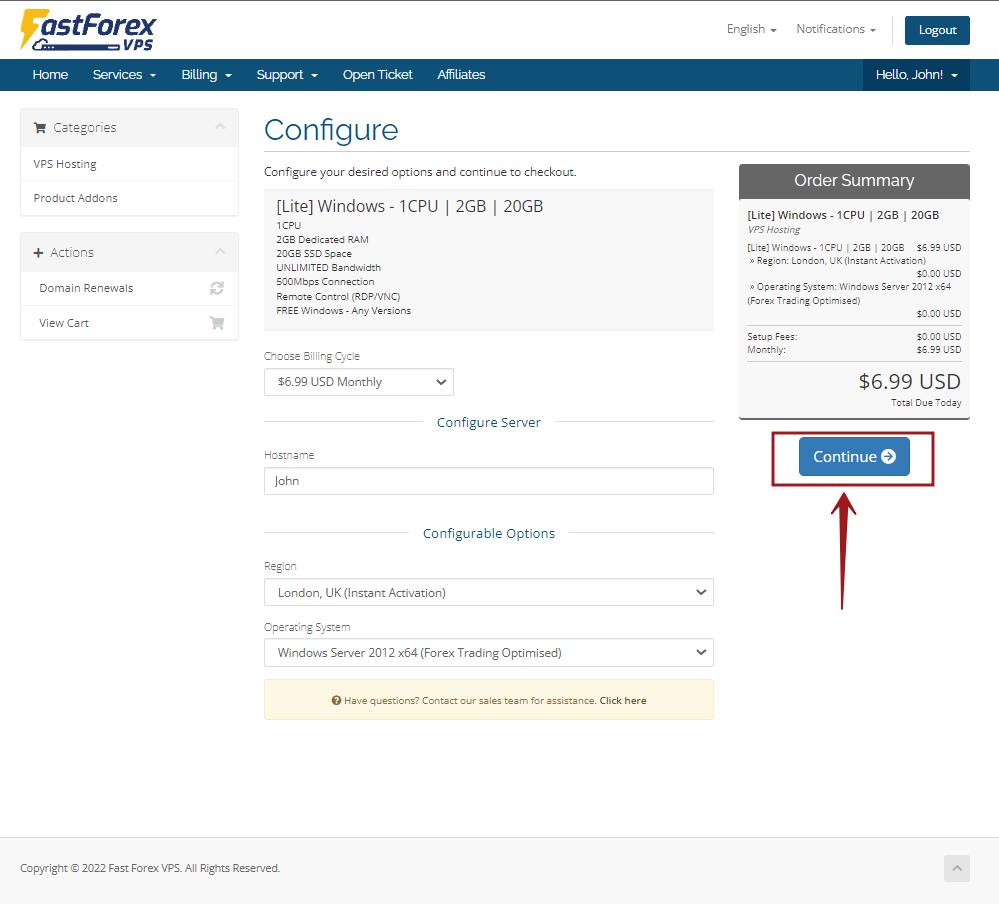In this image, we observe a screenshot set against a solid white background. In the upper left corner, there is a logo for a company named Fast Forex VPS, with the "F" stylized as a yellow lightning bolt. In the upper right corner, there is a logout button. Below these elements, a blue banner menu spans from left to right, featuring options such as Home, Services, Billing, Support, Open Ticket, and Affiliates. On the far right of the banner, there is a pull-down button labeled "Hello John" in white text.

In the center of the image, under the white background, the word "Configure" is displayed prominently in large blue text. Beneath this heading is a gray line, followed by gray text that reads, "Configure your desired options and continue to check out."

To the right side of the image, within a gray box, there is a dark gray banner labeled "Order Summary" in white text. Below this banner, the order details are listed in lighter gray text: "Windows 1 CPU, 2 GB RAM, 20 GB Storage, Monthly Setup Fees," with a total cost of $6.99 USD labeled as "Total Due Today." At the bottom of the gray box, there is a blue action button that reads "Continue."